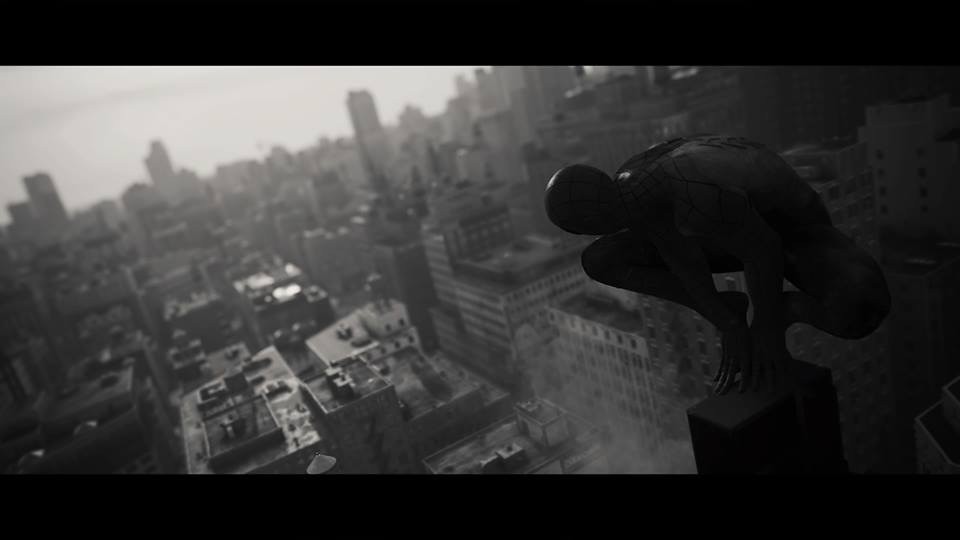This black and white aerial photograph captures a cityscape from a high vantage point, emphasizing the architectural patterns of the city's rooftops. Two black rectangles frame the image at both the top and bottom, providing a striking contrast to the grayscale tones of the city. In the lower right corner, a black viewing platform extends upward from the bottom edge, topped with a distinct half-circle shaped viewfinder. This viewfinder, reminiscent of those often found on observation decks of tall buildings, features a square base and two circular grips on either side, suggesting a tactile experience. The backdrop features a cloudy gray sky, adding to the monochromatic mood of the scene, while the bird's-eye perspective offers a unique glimpse of the city's geometric rooftop layouts.